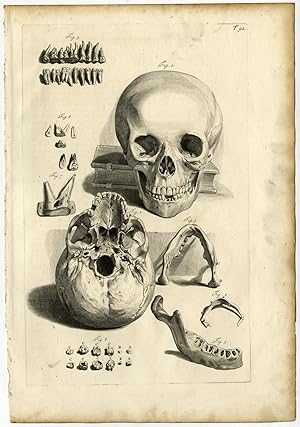This image depicts an aged, tattered piece of paper with a yellowed, brownish tint, suggesting it might be from as far back as the 1950s, if not earlier. The central focus of the drawing is a detailed black and white sketch of a human skull. The main skull is oriented to face the viewer, showcasing typical anatomical features such as a prominent forehead, hollow eyes, a hollow nose cavity, and a partially damaged set of front teeth. Surrounding this central skull are additional illustrations, including another view of the skull from an upside-down angle, which allows a deeper insight into the structure of the mandible and teeth. Throughout the paper, there are detailed drawings of both upper and lower rows of teeth, including molars, bicuspids, and incisors. Individual teeth are also depicted, as well as a jaw detached from the skull. These detailed anatomical sketches suggest the drawing might have been created for medical or dental instructional purposes. The paper itself is notably old and worn, adding to the historical and scholarly feel of the image.